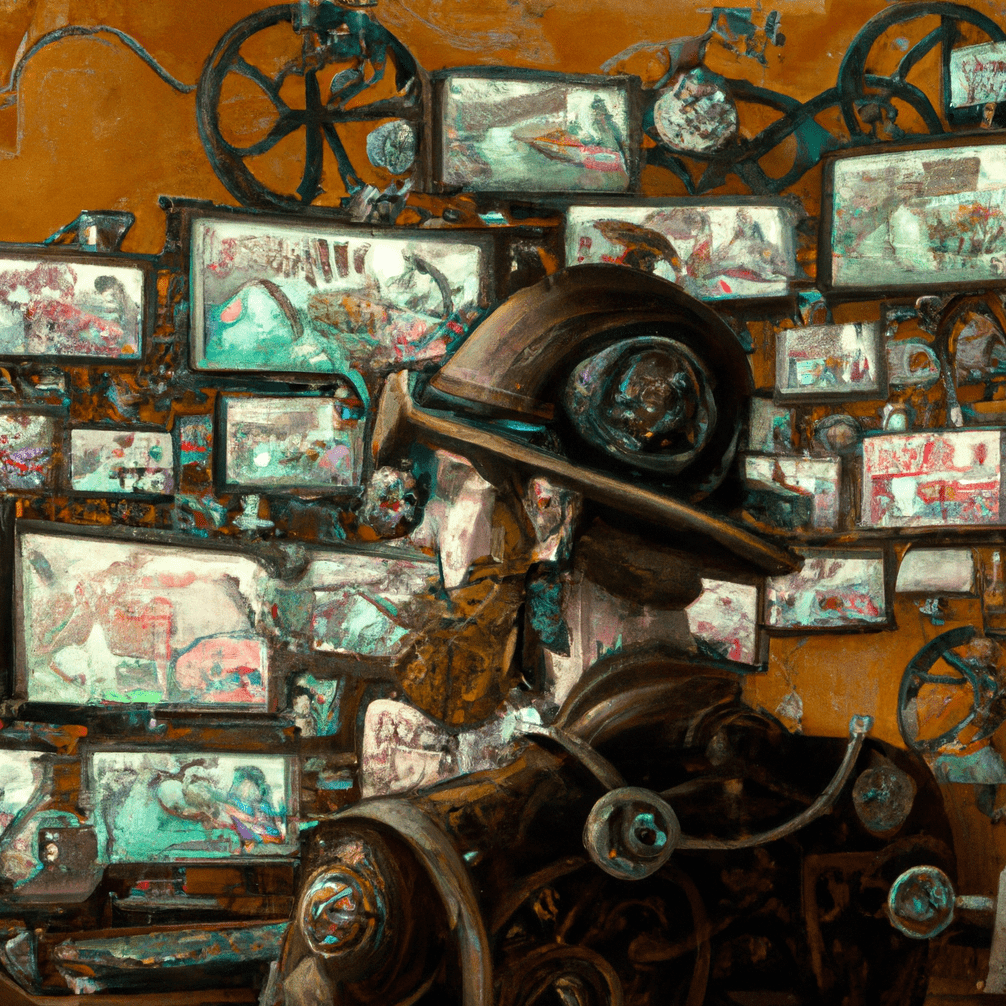The detailed illustration depicts a man with a red beard, wearing a miner's hat adorned with jewel-like patterns and a brownish, mechanical, steampunk-style vest. He stands in front of a large, worn-looking wall filled with numerous rectangular screens of varying sizes, each displaying indistinct images predominantly in blue, red, and green shades. The background of the image is an orange hue, dotted with wheels and intricate mechanical details, enhancing the steampunk vibe. The man, facing the wall of screens with his back towards the viewer, evokes the essence of an old-time explorer or inventor, engrossed in the multiple layers of imagery before him.